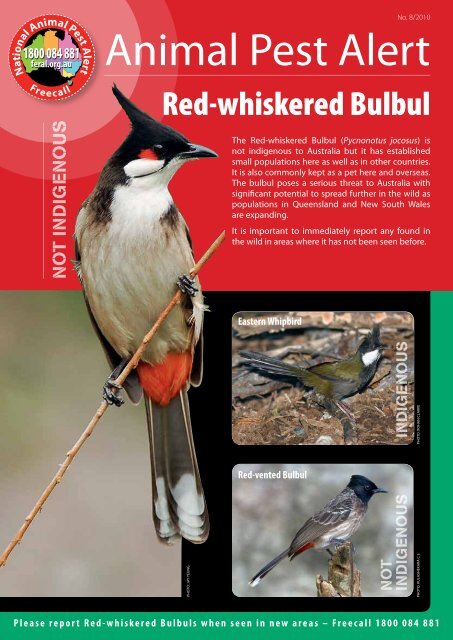The poster is an animal pest alert for the Red Whiskered Bulbul, highlighting its status as a non-indigenous species. The main image showcases the bird clinging to a diagonal branch, displaying its striking appearance: a white chest, a long black beak, and a distinctive crest of feathers atop its head. Its black-gray back contrasts with its black tail and red vent, matching the red spot under its eye. Surrounding this image, the poster features two smaller pictures of similar birds— the Red Vented Bulbul and the Eastern Whipbird. The Eastern Whipbird, which is indigenous, has gray and army green plumage, while the Red Vented Bulbul, also non-indigenous, is gray.

The upper portion of the poster has a red background with large white text declaring the "Animal Pest Alert: Red Whiskered Bulbul." A green border surrounds the entire poster, instructing viewers to report sightings of the Red Whiskered Bulbul in new areas, with a prominent 800 number provided for free calls. Additional text emphasizes the importance of being vigilant about this invasive species and reporting any found, especially in regions where it has previously not been observed. A logo appears on the left, contributing to the official and urgent tone of the message.